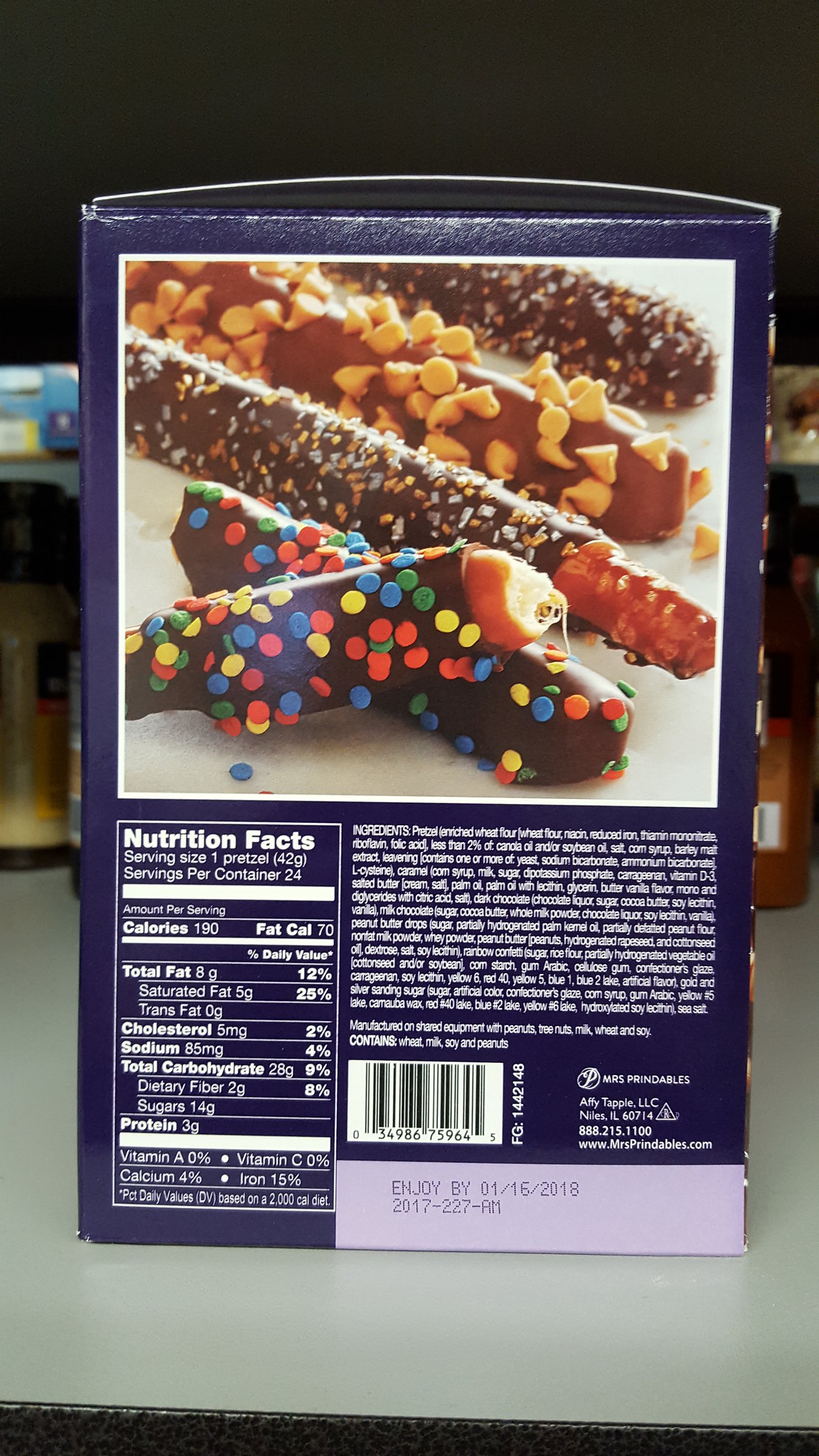The image depicts one side of a product box featuring an assortment of chocolate-covered pretzels. At the top, a vibrant illustration showcases a variety of pretzels intricately coated in luscious chocolate. Two of the pretzels are adorned with small, colorful sprinkles, while another is garnished with butterscotch chips. A unique pretzel topped with round, multicolored dots in green, yellow, and red is also visible, notably broken in two, revealing the crispy interior.

Below the tempting visual, the nutrition facts are clearly displayed. It states that the serving size is one pretzel and there are 24 servings per container. This information is presented on the left side of the box. On the right side, a comprehensive list of ingredients is provided, followed by a distinct UPC code. At the very bottom of the box, the text indicates the best enjoy by date as January 16, 2018, along with a timestamp reading "2017-227-AM."